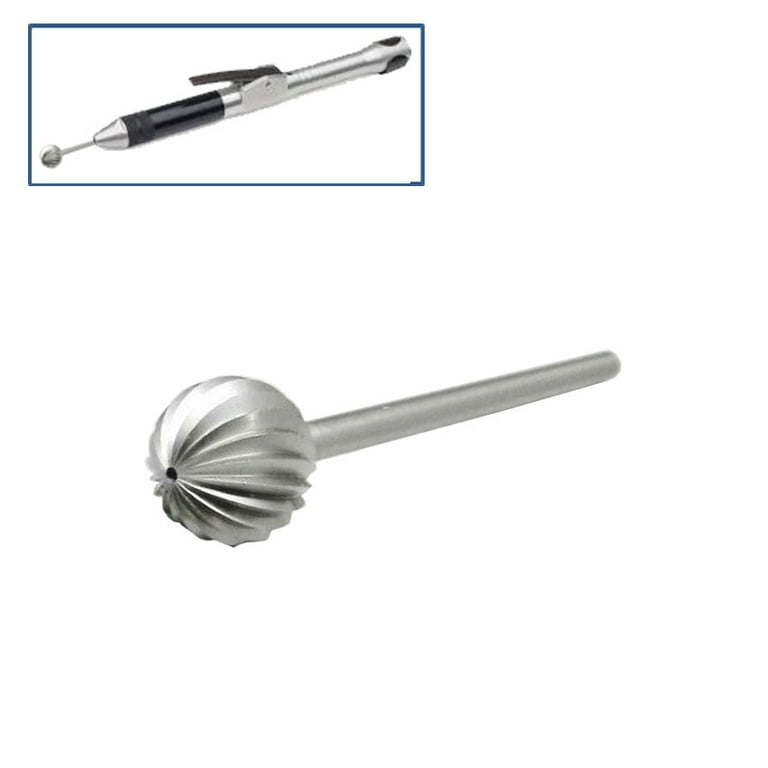The image is divided into two sections prominently set against an all-white background. In the upper right corner, there is a white rectangle outlined with a thin blue line, showcasing a detailed picture of a silver metal tool. This tool resembles a ballpoint pen but features a unique design with a lever situated midway down its shaft. The tool, primarily silver with some black details, extends into a small metal stick at the end where a writing tip would normally be. This stick culminates in a distinctive, textured round ball, which sports deep, vertical ridges running from one pole to the other, similar to a spiraled or ribbed pattern.

Directly below this rectangle, a focused, close-up shot highlights the stick-and-ball component of the tool, amplifying the intricate ridged texture of the ball. The entire tool, viewed in its miniaturized full form and magnified partial detail, exhibits a thoughtfully engineered design, evoking curiosity about its specific functionality.